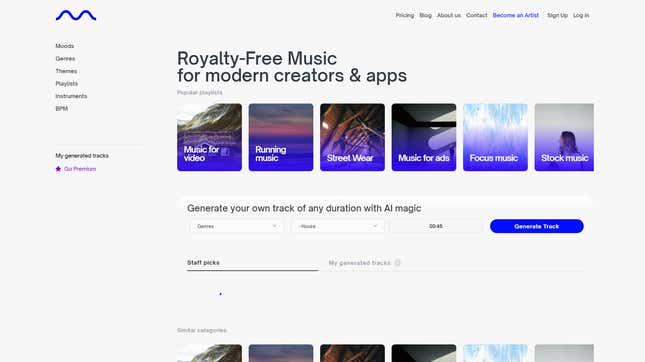The image depicts the homepage of a website dedicated to providing royalty-free music for modern creators and applications. The webpage is primarily designed with a clean, white background and black text, complemented by accents of purple in various elements. 

At the top of the page, a prominent headline reads, "Royalty-Free Music for Modern Creators and Apps," setting the tone for the site's offering. Below this headline, there are six equally spaced squares aligned horizontally, each featuring a different image and a purple bottom border with white text overlay.

1. The first square features a rugged, rocky mountain landscape and is labeled "Music for Video."
2. The second square shows a serene sunset background with the label "Running Music."
3. The third square includes an image of a musical instrument or a street scene, simply labeled "Music."
4. The fourth square's image is indistinct, but it is labeled "Music for Ads."
5. The fifth square reminds one of rainfall and is labeled "Focus Music."
6. The sixth square displays a profile picture of a girl with long blondish hair, labeled "Stock Music."

Directly beneath these squares, there is a line of black text that reads, "Generate your own track of any duration with AI magic." To the right of this text, a large purple oval button is prominently displayed, labeled "Generate Track," inviting users to create their own music.

This descriptive and visually engaging webpage layout is designed to cater to the needs of modern content creators seeking high-quality, royalty-free music solutions.